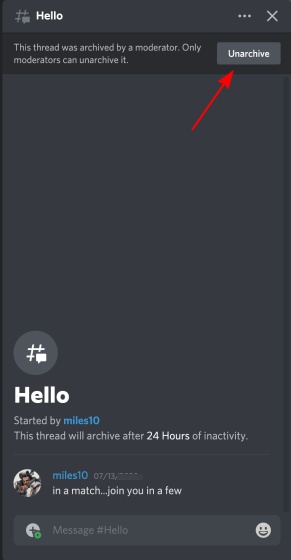A screenshot captures an ongoing conversation on a website or app, possibly involving customer support. The interface is primarily in dark grayscale tones. At the top of the page, a graphic features a hashtag and a small message box with the bold white text “HELLO.” Below this, in smaller text on a darker background, it states that the thread was archived by a moderator, with a red arrow pointing to an "UNARCHIVE" button – highlighting the thread's status and the undo option.

The conversation appears to be minimal, initiated by a user named "miles10," whose name is highlighted in blue. There's an avatar of miles10 and the timestamp "July 13." The next line reads, “This thread will archive after 24 hours of inactivity.” Miles10’s message states: "In a match, join you in a few." 

At the bottom of the screen, there's a message bar prompting the user with "You can message #hashtag," accompanied by an option to add emoticons. The interface seems prepared for further interaction despite the current archival status of the thread.